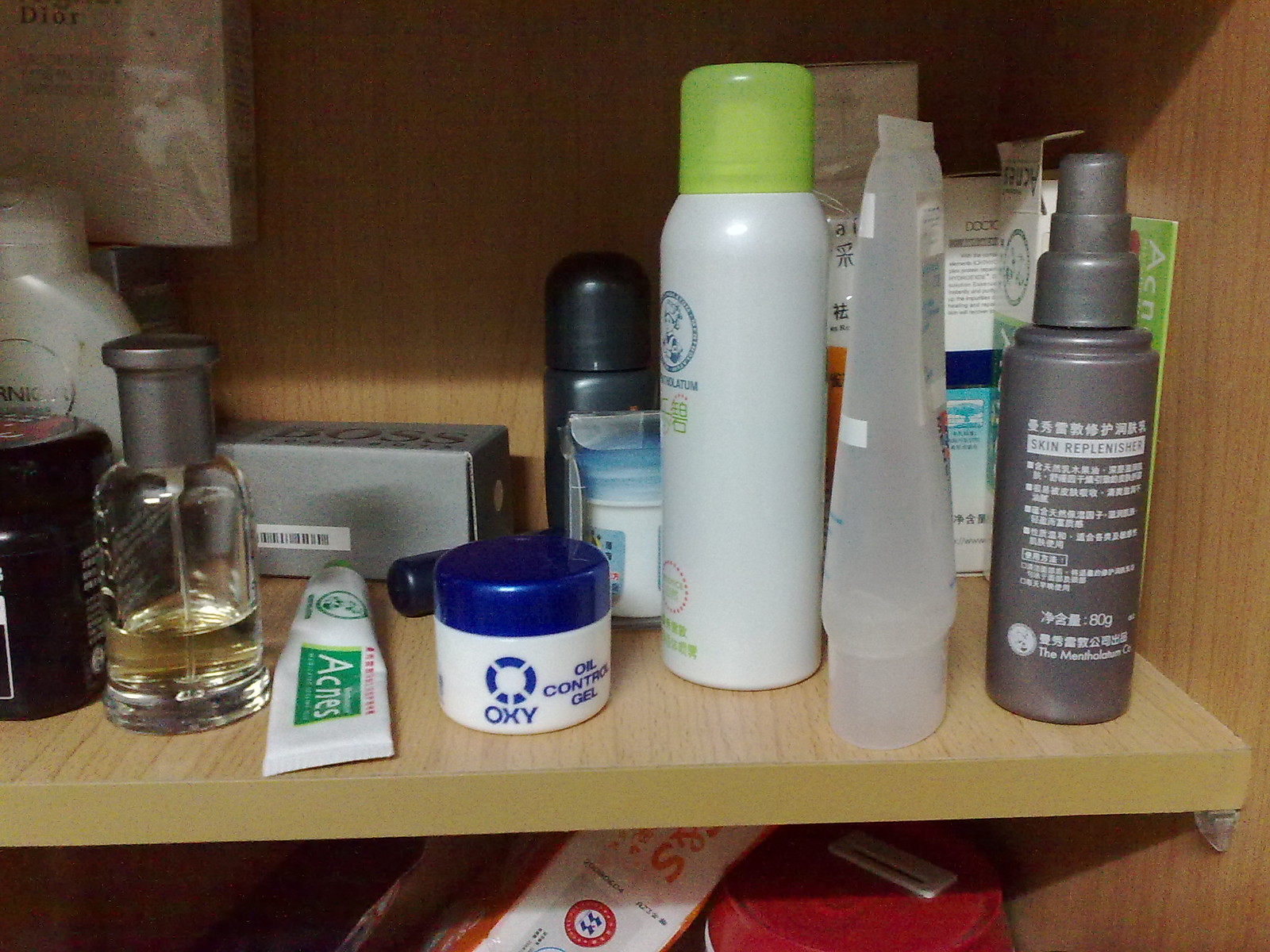The photograph depicts a cluttered assortment of personal care items arranged on two shelves within a blonde wood cabinet. On the bottom shelf:

- A white bottle of lotion with a matching white lid.
- A sleek black container adorned with white text.
- A clear glass bottle capped with a gray lid.
- A gray box featuring dark font and a visible barcode.
- A white tube with green and white detailing.
- A round, white, and blue container positioned in front of a black object.
- Another white and light blue container, slightly obscuring a dark gray container behind it.
- A white bottle with a green lid positioned prominently at the forefront.
- A clear plastic container with blue font etched on its surface.
- A gray spray bottle labeled in white font.
- Visible in the background are a green card, a white box, a white and blue box, and a yellow and gold object.

On the second shelf:

- An object with a red lid.
- A box featuring multiple colors: red, blue, black, and orange.

The overall image quality is grainy, adding a tactile and somewhat nostalgic texture to the scene.